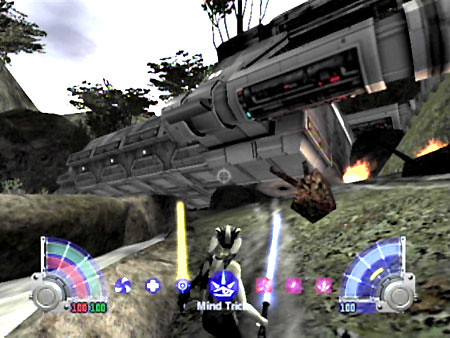This detailed screenshot from a video game showcases a futuristic scene featuring a robotic device resembling a spaceship. The sleek, gray apparatus, adorned with doors and lights, hovers in the sky. Below the device, small flames flicker ominously. The background reveals the tops of lush green trees set against a vivid blue sky dotted with wispy white clouds.

In the foreground, we see the back of a character that appears to be a hybrid of human and animal, identifiable by their distinct white hair and animal-like ears. The character is armed with a glowing yellow sword held in their left hand. The scene is alive with vibrant lights, adding a dynamic and immersive quality to the image.